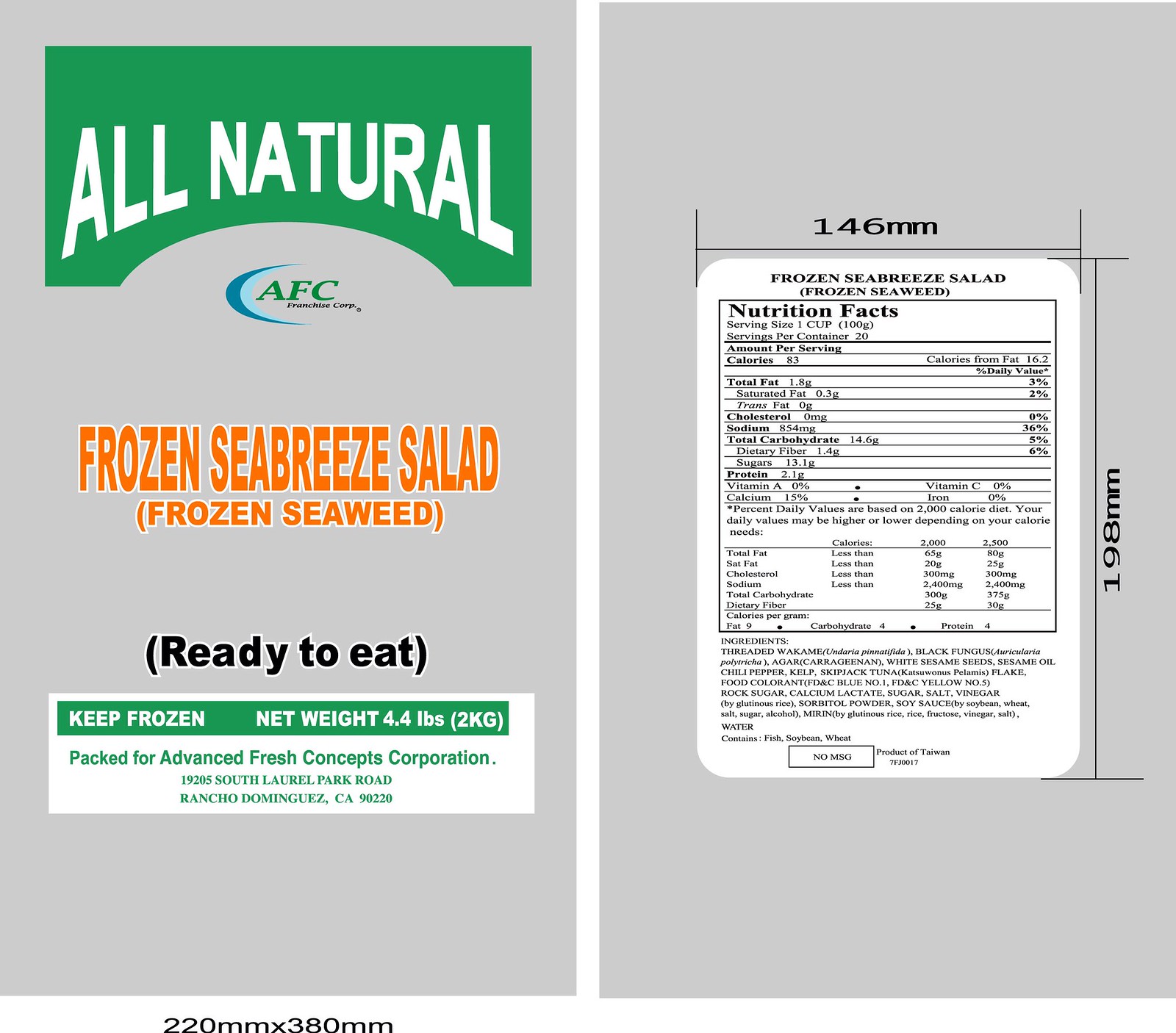The image is a dual-picture preview of a salad bag's packaging, split into two distinct sections positioned side by side. The left section showcases the front label of the bag. At the top, it prominently features the phrase "All Natural." Centrally displayed is the product name: "Frozen Sea Breeze Salad: Frozen Seaweed." Below this, the label indicates that the product is "Ready to Eat" and should be "Kept Frozen." The packaging information specifies that it is "Packed for Advanced Fresh Concepts Corporation." The bottom of the left section includes measurement markings, possibly for dimension reference.

The right section of the image displays the Nutrition Facts label in black and white. This label provides detailed nutritional information, listing key components such as Total Fat, Cholesterol, Sodium, Sugars, Proteins, and various Vitamins. It also enumerates the Ingredients used in the salad. Alongside the Nutrition Facts table, there are measurements denoting the Height and Width of the label, providing clear dimension specifications. This detailed portrayal offers a comprehensive look at both the branding and nutritional information available on the salad bag's packaging.